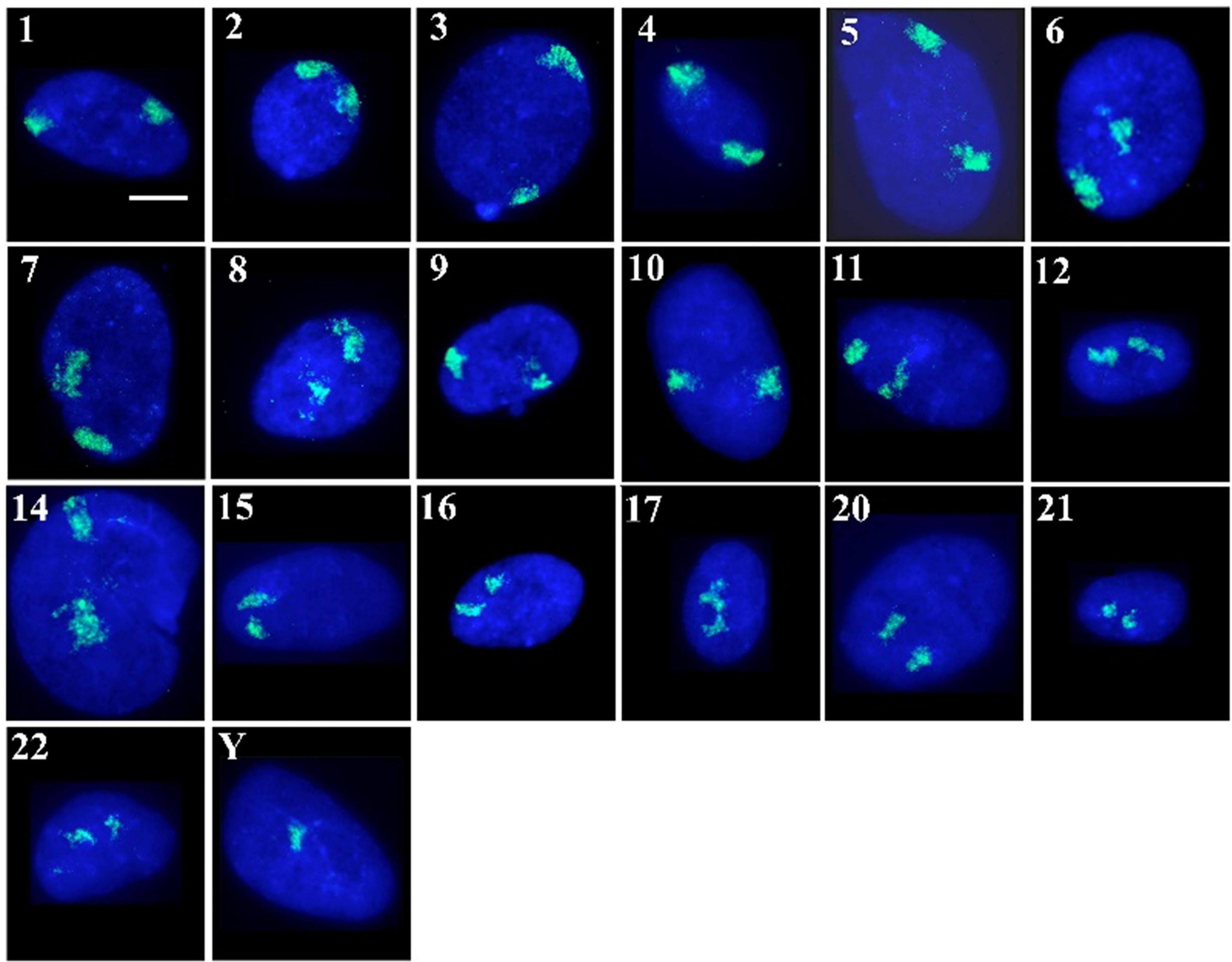This photograph showcases a grid of 23 squares, arranged in a black background, each numbered consecutively from 1 to 22, with the final square labeled 'Y'. The images appear to be microscopic photos featuring blue oblong or oval-shaped objects, each highlighted with patches of light green. Each object seems to possibly represent the same item but captured from different viewpoints or variations. The images are illuminated, giving a glowing effect, particularly evident due to the laser-like blue light. Notably, all squares maintain uniformity with the black backdrop and numbered white labels in the upper left corner, except for the last square 'Y', which uniquely contains only one light green spot in its center. The absence of any additional labels, titles, or identifying information such as time, date, or specific names of the species, contributes to the enigmatic nature of the image.